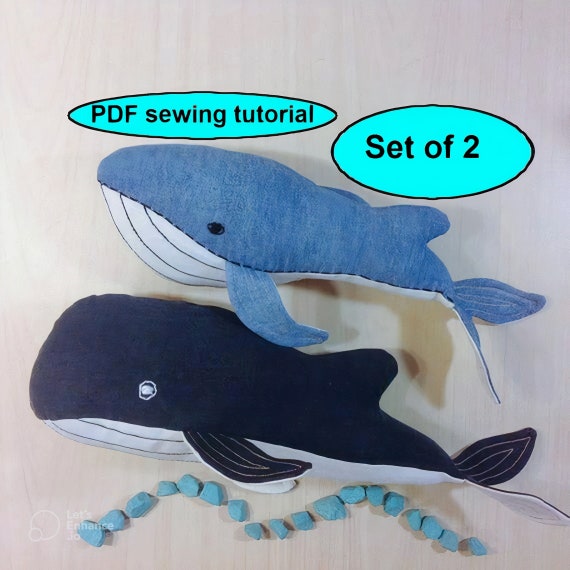This web advertisement photograph features two meticulously hand-sewn stuffed whales positioned at the center, set against a textured, light tan wood background. Both whales, one a lighter blue and the other a dark navy, display detailed white stitching along their undersides, intricately embroidered fins, tails, and black or white sewn eyes. The top of the image includes two computer-generated bubbles with a black font on an aqua background; one reads "PDF Sewing Tutorial" while the other states "Set of Two." These whimsical whales rest atop a wave pattern crafted from small blue stones, enhancing the image's aquatic theme. An opaque logo in the bottom left corner reads "Let's Enhance Joe," adding a subtle branded touch.